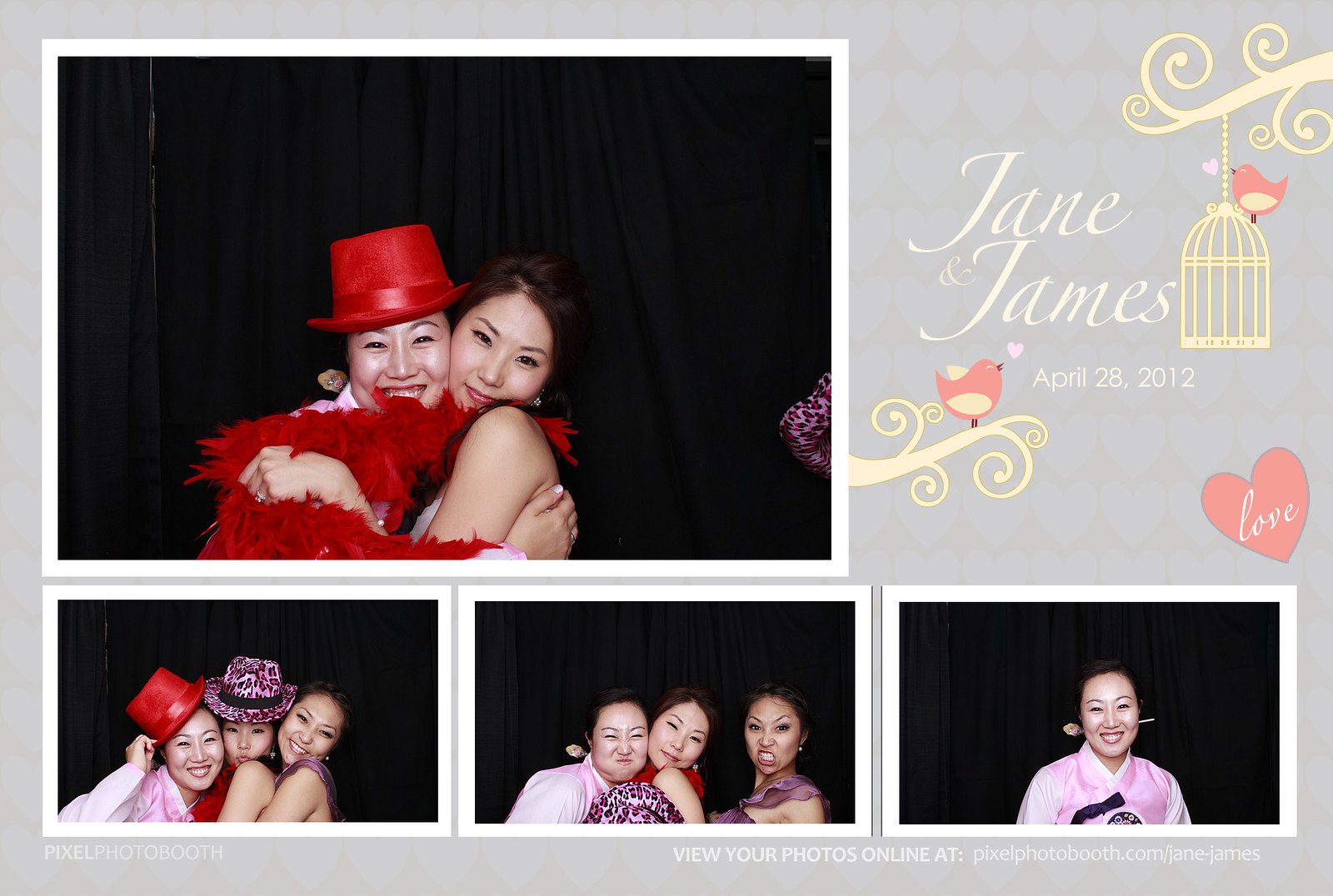This image is of a greeting card with a detailed, collage-like design. The background is predominantly blue with light gray hearts scattered like watermarks, complemented by swirly golden branches at the top right and bottom left, each adorned with a bird and a small pink heart emanating from their mouths. At the center, the names "Jane and James" are elegantly displayed in white, alongside the date "April 28, 2012." Below the text, there is a collage comprising four photographs set against a black curtain backdrop. 

The top photograph features two young Asian ladies, one in a pink dress with a red hat and scarf, being hugged by another girl in a sleeveless dress. They smile at the camera while an elbow of a third person is slightly visible. Three smaller photographs are lined underneath: the first shows three girls, with one holding the red hat and another wearing it, all posing playfully. The second image captures the same trio, making various faces for the camera without the red hat. The third and final image on the right focuses on the girl in the pink and white traditional Japanese attire, smiling directly at the lens. 

Footnotes at the bottom of the card read "pixel photography photo booth" and a link to view online photos: "pixelphotobooth.com/jane-james."